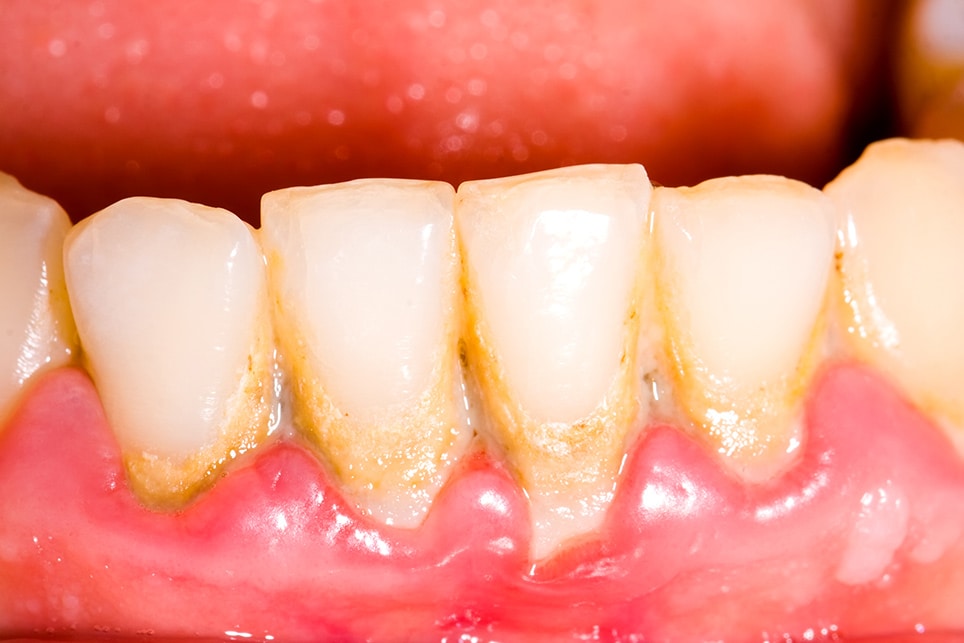This image is a highly detailed close-up of a person's lower front teeth, specifically showcasing six visible teeth along with the gum line and part of the tongue blurred at the top. The teeth are in poor condition, displaying a significant buildup of yellowish-brown plaque and darker greenish tartar at the base and between the teeth, suggesting extensive neglect. In some areas, the buildup appears black and gray. The gums are notably inflamed, swollen, and exhibit a pronounced redness, particularly in the center, indicating possible gum disease. There are also white spots on the gums, possibly canker sores, as well as smaller, lighter pink spots on the lower left side. The teeth themselves are jagged and not well-maintained, with the central two teeth slightly taller than the others. Overall, the image reveals significant dental and gingival issues that likely require professional cleaning and care.